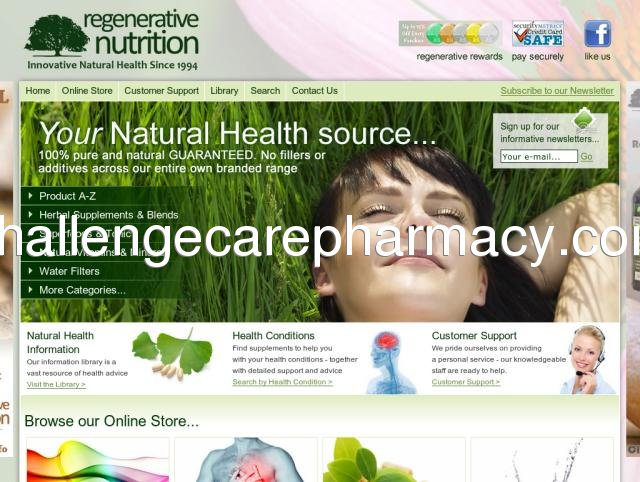In the upper left corner, a vibrant image of a large green tree stands out, accompanied by the text "Regenerative Nutrition." Beneath this, the phrase "Innovative Natural Health Since 1994" is prominently displayed. Below, a serene image of a woman lying peacefully in lush green grass is showcased. The woman has dark brown hair, her eyes are closed, and she appears utterly relaxed and content. Beside her, the text reads, "Your Natural Health Source… 100% Pure and Natural Guaranteed. No Fillers or Additives Across Our Entire Branded Range."

In the upper right corner of the image of the woman, there is a call to action: "Sign Up for Our Informative Newsletters," along with a designated area for entering an email address. Below this section, various subcategories are presented. "Natural Health Information" is listed alongside an image of green leaves. "Health Conditions" is illustrated with an image highlighting the brain in red and the neck and face in blue. Additionally, "Customer Support" is depicted with an image of a woman wearing an earpiece and microphone, ready to assist.

At the bottom, the text "Browse Our Online Store" invites viewers to explore further, highlighted by bright rainbow colors in the bottom left corner. The main website information is displayed in white text: "www.allengecarepharmacy.com."